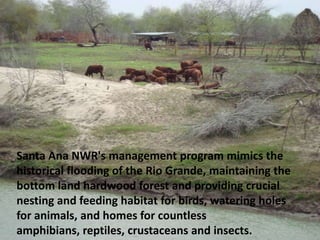The image depicts a small, vibrant farm or ranch set against a lush, green landscape. Prominent features include verdant grass fields, sporadic dry patches, and clusters of trees, likely oak, with brown branches. Scattered across the grassy expanse are grazing animals, potentially sheep, goats, or cattle, though their exact species is indiscernible due to the blurry quality. In the middle distance stands a barn or similar structure, situated near the bank of a flowing river, adding to the rustic charm. Above, the sky is clear with shades of blue, enhancing the picture's pastoral ambiance. A text overlay at the bottom of the image, in black lettering, reads: "Santa Ana NWR’s Management Program mimics the historical flooding of the Rio Grande, maintaining the bottomland hardwood forest and providing crucial nesting and feeding habitats for birds, watering holes for animals, and homes for countless amphibians, reptiles, crustaceans, and insects." This text emphasizes the environmental efforts in maintaining the natural habitat and biodiversity of the area.